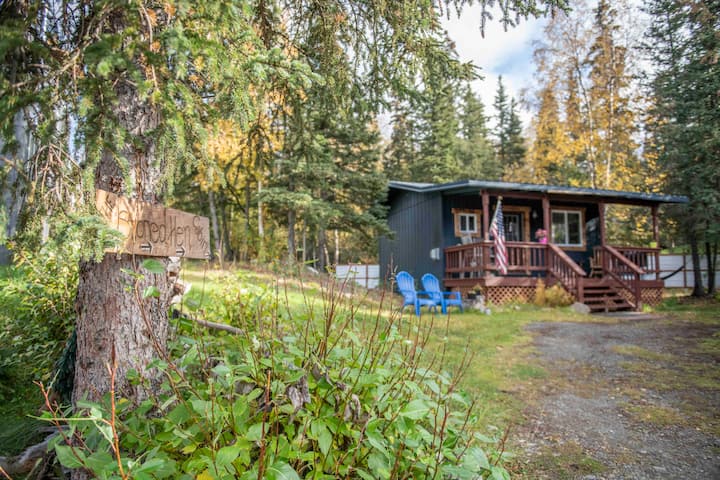The photograph captures a small, dark gray cabin set in a rural area, surrounded by a multitude of tall evergreen trees under a blue sky with scattered white clouds. The cabin, featuring a brown wooden porch and a gray roof, has an American flag hanging from a pole attached to the porch. A dirt pathway leads up to the front steps of the cabin, where a simple door is flanked by one window to the left and a smaller window to the right. Adjacent to the cabin, on its left side, are two blue Adirondack chairs. In the foreground, to the left of the frame, a large tree trunk stands closer to the camera with a wooden sign attached, bearing text that reads "The Hen Cabin" or similar. Below the sign, a bushy area with prominent gray sticks can be seen. The expansive greenery surrounding the cabin hints at a serene, secluded setting.